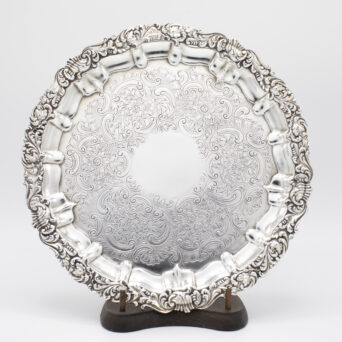This square image features a decorative plate standing on a dark wooden base with two vertical pegs. The backdrop is a light gray shade, enhancing the focus on the ornate object. The wooden stand has a dog bone or kidney shape, providing a sturdy support for the plate.

The plate itself is a silver color with a textured and intricately engraved design around its edges, consisting of curved lines and swirls, akin to floral and banner-like patterns. The rim is adorned with an elaborate, ornate design. The center of the plate features a distinct white circular section. This central area isn't plain; it appears almost cutout, flaunting additional subtle designs that might be painted on or result from the high polish or wear, giving it a complex, textured look. The white central portion might also have bumps and dots as part of its intricate detailing. The plate stands vertically on the wooden pegs, facing the observer directly, showcasing its rich detailing and craftsmanship.